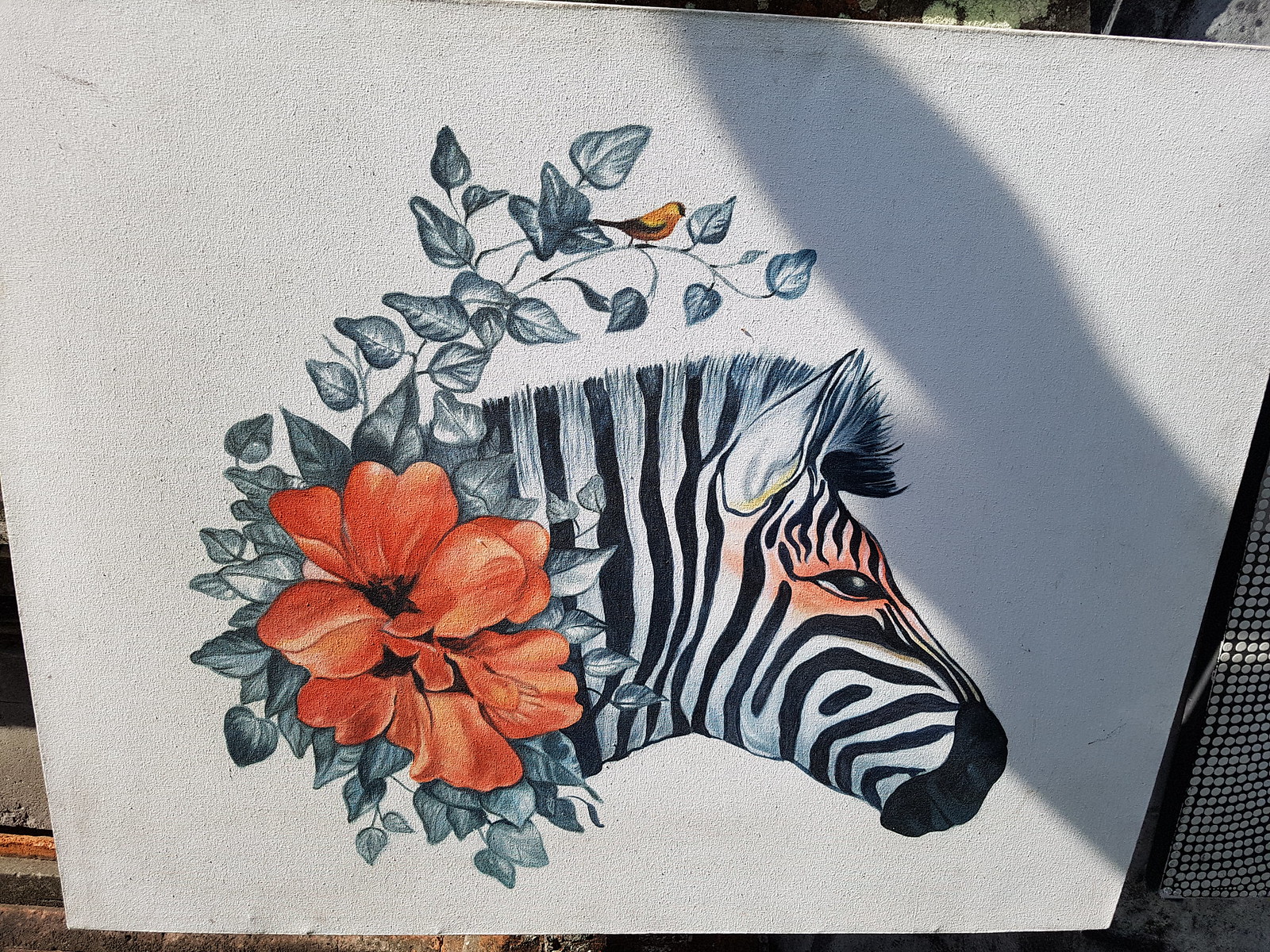A vibrant color photograph captures a striking drawing displayed on a white sketch pad, positioned upright and slightly leaning against an unseen support. The artwork features the head of a zebra, meticulously illustrated with what appears to be a combination of colored pencils, inks, or perhaps paint. The zebra's monochromatic black and white stripes contrast beautifully against the surrounding vivid elements. A bold red hibiscus flower, accompanied by lush green leaves, adorns the area where the zebra's neck would extend, forming a wreath-like frame around the head. Adding to the enchanting scene, a small bird is intricately depicted emerging from the leafy arrangement, enhancing the whimsical, illustrative quality of the piece. The photograph effectively captures the essence of the drawing, which could easily serve as an illustration for a storybook.